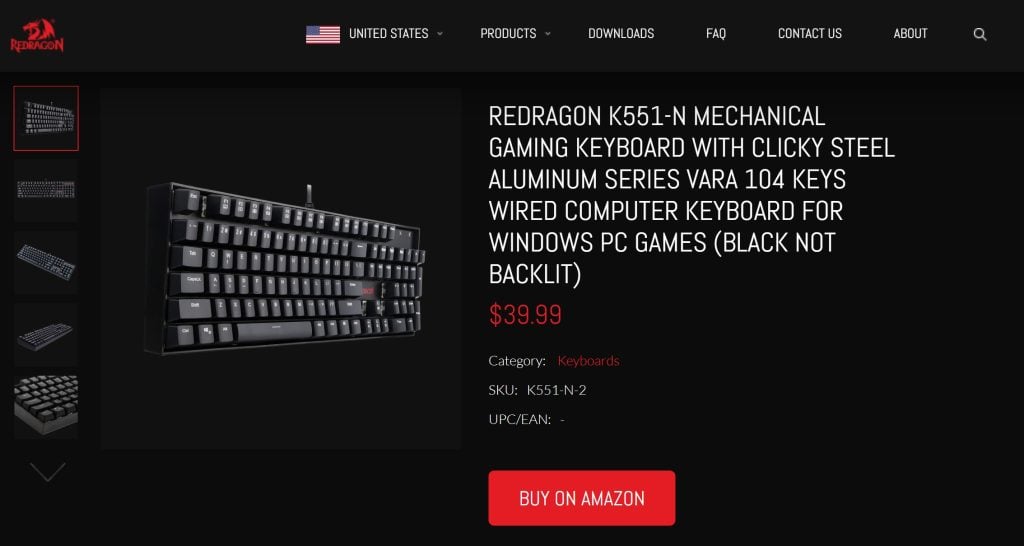This is an Amazon advertisement page specifically for the American market, as indicated by the prominently displayed American flag. The seller’s name is unclear, but their red logo and red text are visible. The advertisement features an image of a locker with numerous small drawers, suggesting a wide variety of items for sale. 

In the center of the screen, the product being highlighted is the "Red Dragon K551-N Mechanical Gaming Keyboard." The keyboard is part of the "Clickity Steel Aluminium Series Vara" and features 104 keys. It is designed as a wired computer keyboard for Windows PC games, available in a black color but notably not backlit. The price of the keyboard is prominently displayed in red as $39.99. The product falls under the category "Keyboards," with an SKU of "K551-N-2." Additionally, there is a mention of "UPC/EAN," although the numbers are not specified. A conspicuous red button labeled "Buy on Amazon" invites potential buyers to make a purchase. The entire advertisement is set against a black background, giving it a dark and sleek appearance.